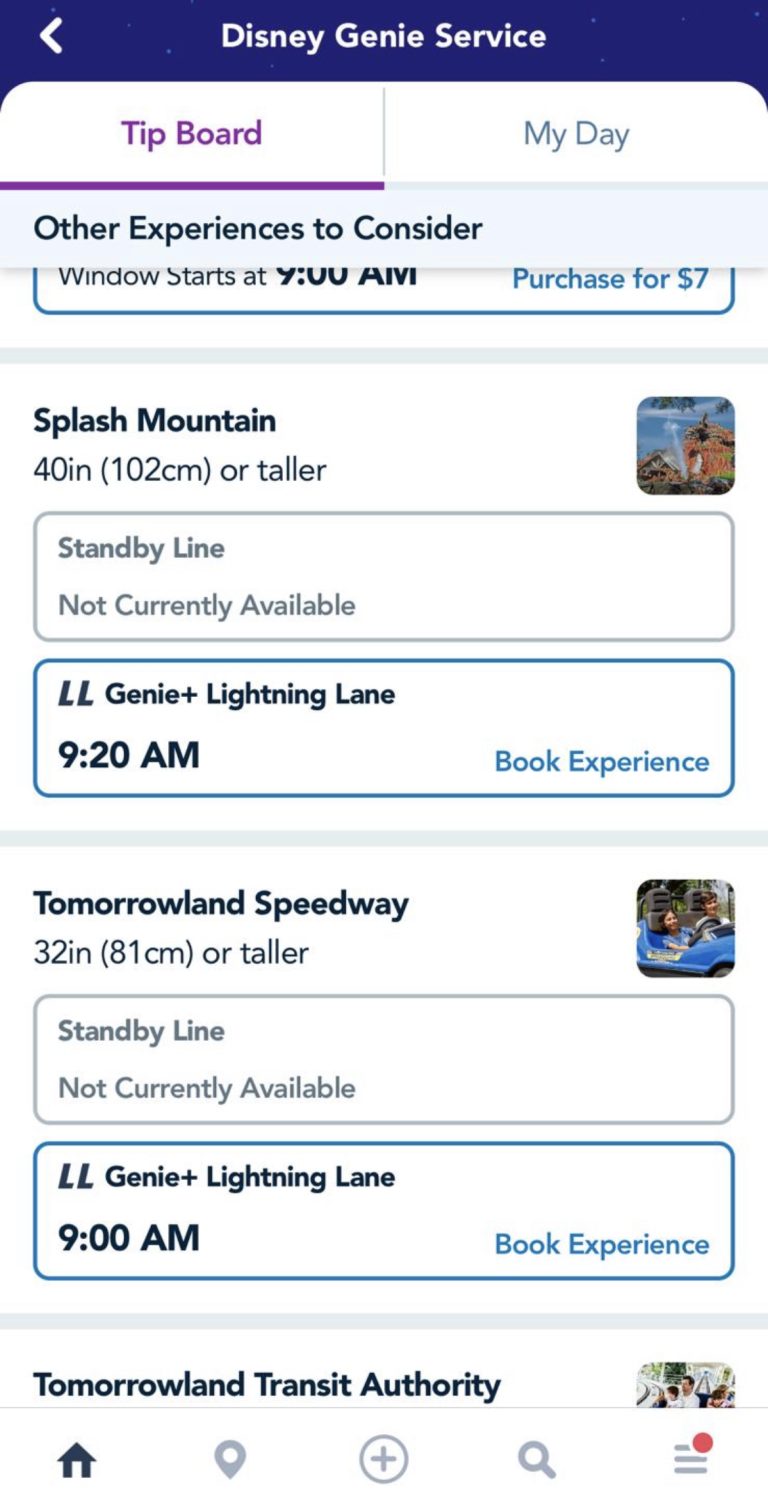The image displays a Disney Genie+ service interface. The header section of the image features white text on a blue background, stating "Disney G9 Service." Below the header are two tabs: "Tip Board" on the left and "My Day" on the right. "Tip Board" is highlighted in purple, indicating it is the active tab, while "My Day" is blue.

Immediately beneath the tabs, there is black text that reads, "Add experiences to continue." Following this, another section of text states, "Windows start at 9:00 a.m. Purchase for $7," with "Purchase for $7" highlighted in blue.

The first highlighted section showcases Splash Mountain. It specifies height requirements of 40 inches (102 centimeters) or taller. There is a note that the standby line is not currently available. Two options are listed: "Genie+ Lightning Lane 9:20 a.m. Book Experience," with "Book Experience" highlighted in blue, signifying it is clickable. This section is outlined in blue, indicating selection, and a small picture of Splash Mountain is on the right.

The second highlighted section details Tomorrowland Speedway with a height requirement of 32 inches (81 centimeters) or taller. Similar to Splash Mountain, the standby line is not currently available. The option presented is "Genie+ Lightning Lane 9:00 a.m. Book Experience," with "Book Experience" highlighted in blue. This section is also outlined in blue, indicating it is selected.

Overall, the interface guides the user through the process of booking experiences via the Genie+ service, providing clear options and visual selection indicators.